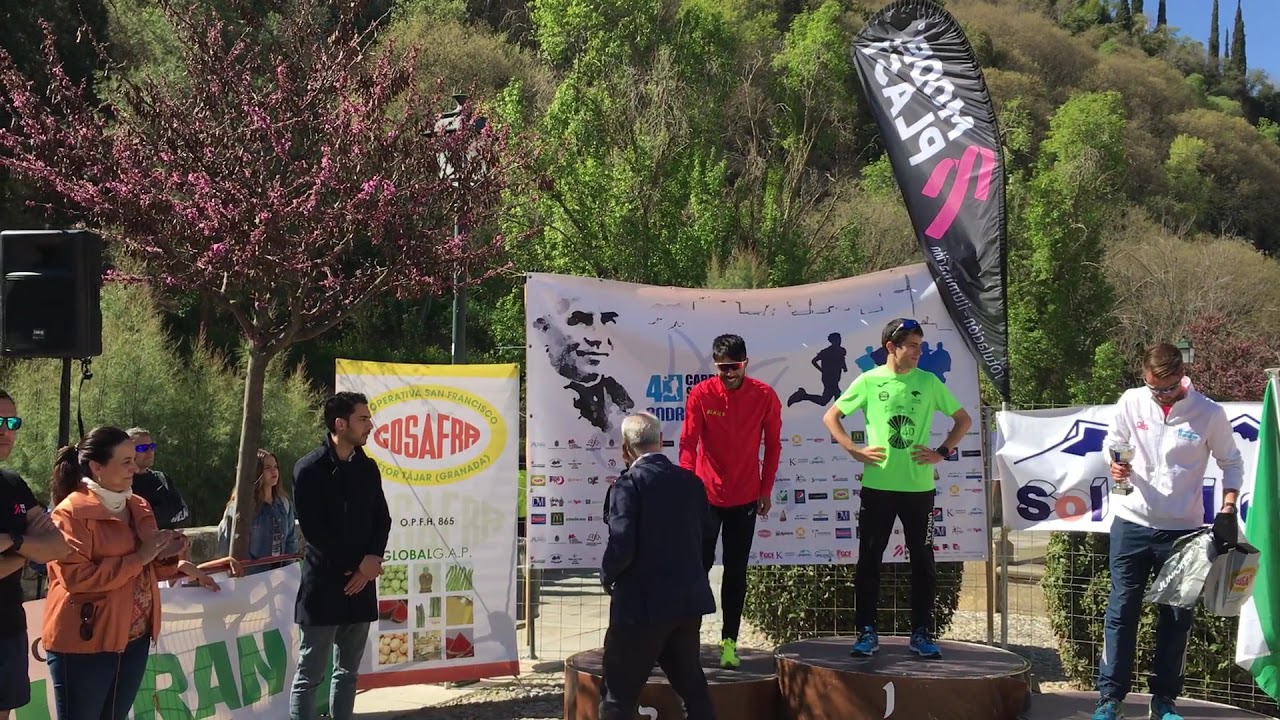The image captures an outdoor awards ceremony, likely celebrating a running or jogging event. At the center of the image, there are rounded, brown podiums, with the highest podium labeled "1" occupied by a man towards the middle right. This man, standing in a victorious stance, is dressed in a lime green shirt, black pants, and blue running shoes, with his hands on his hips and sunglasses resting on top of his head. To his left, another man stands on a lower platform, wearing a red long-sleeved shirt, black pants, and sunglasses. In total, there are about nine people in the image. Various banners advertising different sponsors are visible behind them, set against a backdrop of trees displaying a mix of purple and green foliage. A hillside rises in the background, adorned with trees and bushes, and is equipped with electronic gear for broadcasting, including a display screen. On the right side, a man in a white sweater and blue jeans holds a trophy and several bags. The event appears to be taking place in a foreign country, as indicated by the unfamiliar language on the banners. Spectators can be seen on the left side of the image, along with a speaker positioned above the participants' heads.